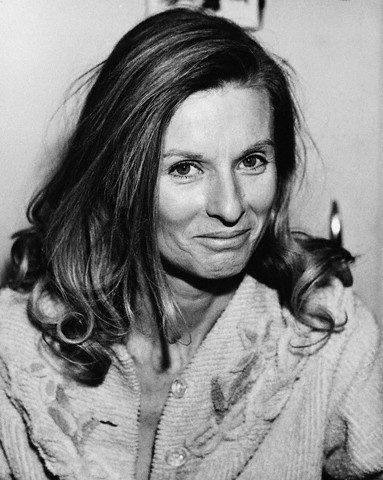This image is an old black-and-white photograph of the renowned actress Cloris Leachman, likely taken in the 1960s when she appears to be in her 30s. She gazes directly at the camera with the beginning of a smile playing on her lips, her expressive eyes twinkling with a hint of warmth and playfulness. Her long hair, characterized by dark strands with lighter streaks, is parted to the side and cascades past her shoulders, curling slightly at the ends. 

Leachman is dressed in a textured jacket that resembles corduroy or terrycloth, adorned with clear plastic or glass buttons, several of which are undone, revealing her neck and the upper part of her chest without exposing her breasts. The jacket also features subtle patterns that might be floral or leafy, adding a touch of intricacy to her appearance. 

The background is a plain white wall, ensuring that all attention is drawn to Leachman's striking presence in this close-up portrait that captures her head and torso. One can also discern a small, square object on the wall above her head, though its details are not distinct.